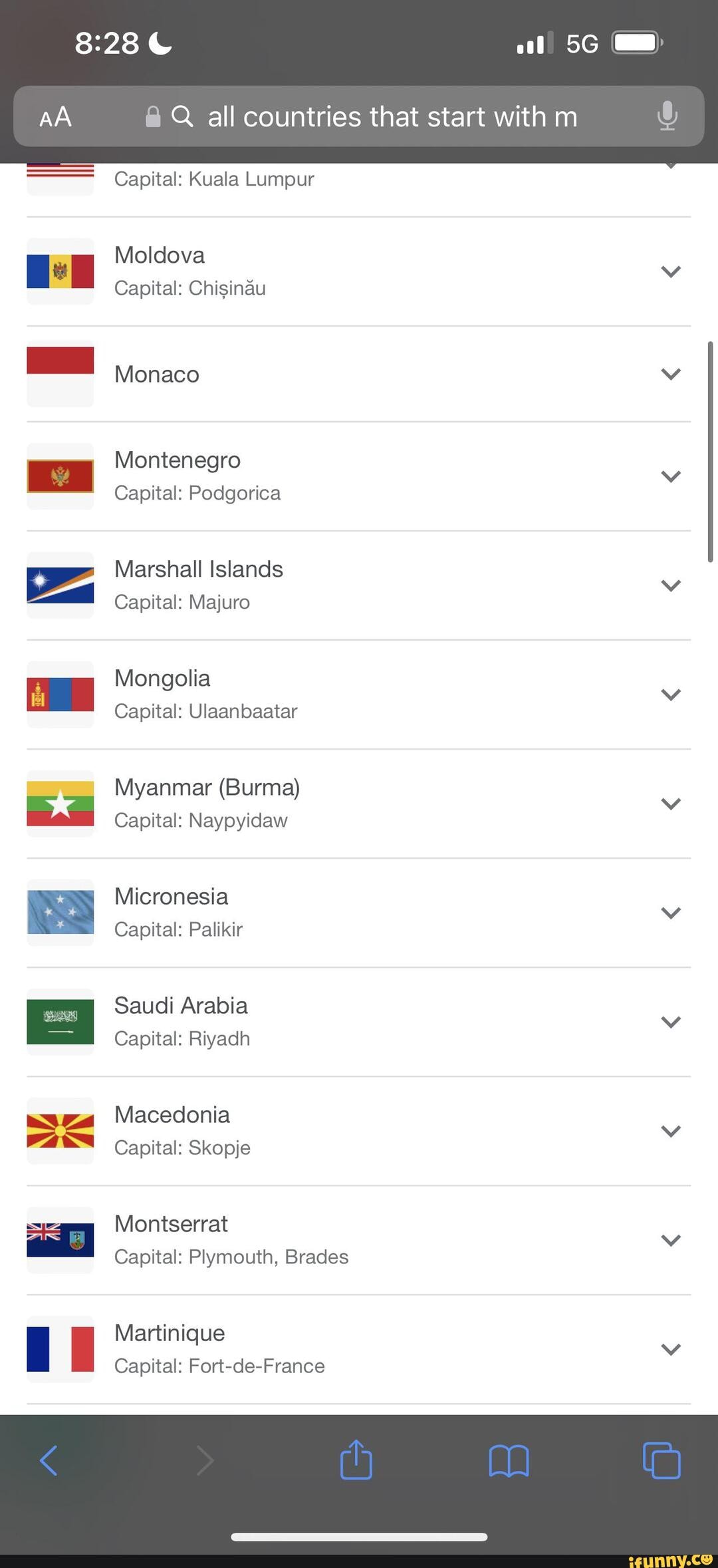Certainly! Here's a detailed and cleaned-up caption for the described image:

---

A screenshot from a cell phone displays several details along with a list of countries. The top of the screen features a black header showing the time '8:28', accompanied by a crescent moon icon. To the right of the header, there are three lit bars out of four indicating signal strength, a '5G' label, and a full battery icon. Below this header is a grey search bar with the text 'Countries that start with M'. The main section of the image displays a list of countries on a white background, each separated by thin grey horizontal lines. The countries listed from top to bottom are:

1. **Moldova** - Capital: Chisinau
2. **Monaco** - Represented with a red and white flag
3. **Montenegro** - Capital: Podgorica
4. **Marshall Islands** - Capital: Majuro
5. **Mongolia** - Capital: Ulaanbaatar
6. **Burma (Myanmar)** - Capital: Naypyidaw, shown with a yellow, green, and red striped flag with a white star in the center
7. **Micronesia** - Capital: Palikir

---